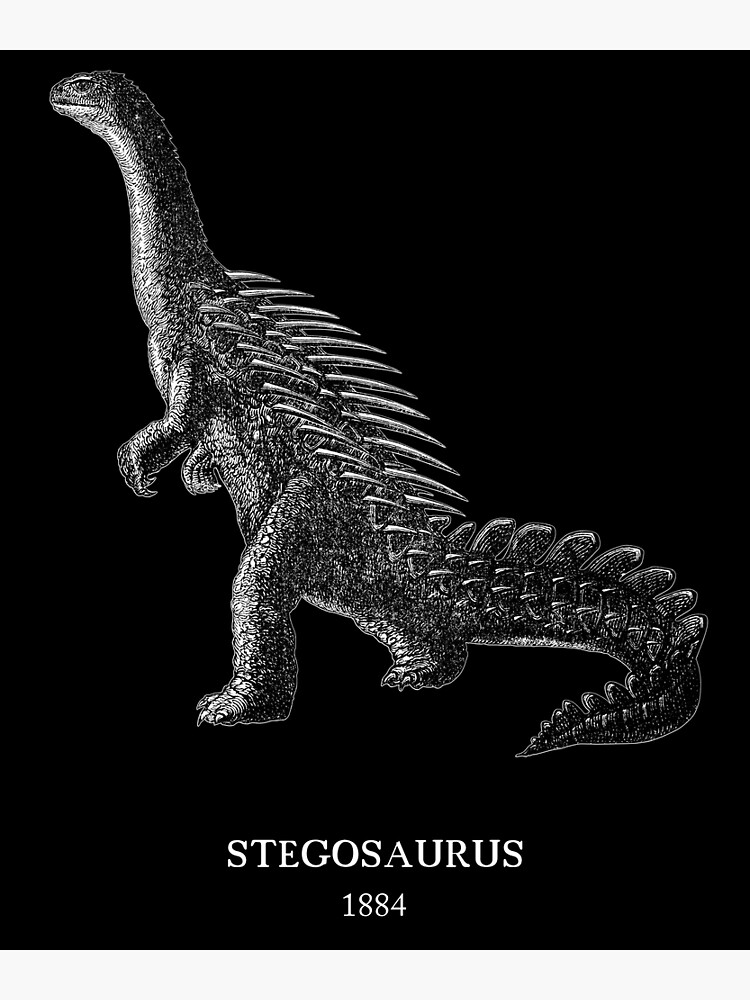This detailed black and white illustration from 1884 depicts a Stegosaurus against a completely black background. The dinosaur is portrayed standing on its muscular hind legs, with noticeably shorter front legs that are equipped with small claws. Its long neck extends gracefully, adding to its imposing stature. The tail is reminiscent of a crocodile's, appearing quite heavy and armored, and features fin-like structures. Along its back, a series of porcupine-like spines or tusks are prominently displayed. The Stegosaurus is facing left in the image, which may have served as an advertisement. The overall impression of the creature is one of strength, with a mix of crocodilian and spiny features enhancing its prehistoric mystique. The dinosaur and its background are rendered in shades of black, white, and gray, with the text “Stegosaurus 1884” clearly visible at the bottom.